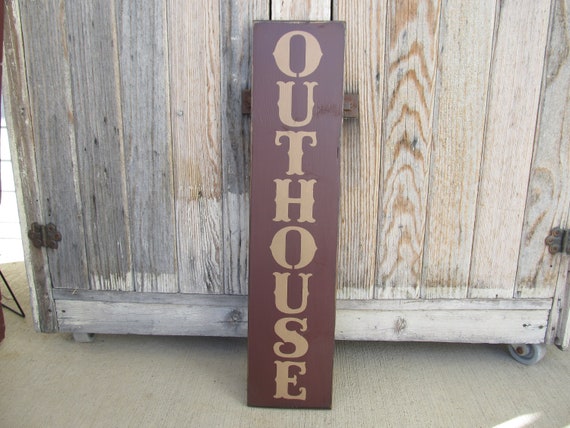This photograph captures a long, narrow brown sign with the word "OUTHOUSE" written vertically in capital letters with a gold or beige font. The sign, which exudes a vintage charm, is leaning against a light brown wooden structure that resembles a cabinet on wheels. The cabinet, showing signs of age and wear with rusted dark brown hinges, rests on gray casters. The surrounding floor appears to be wooden but lighter in color and less rustic. In the left portion of the image, there is a hint of a wire or metal stand.